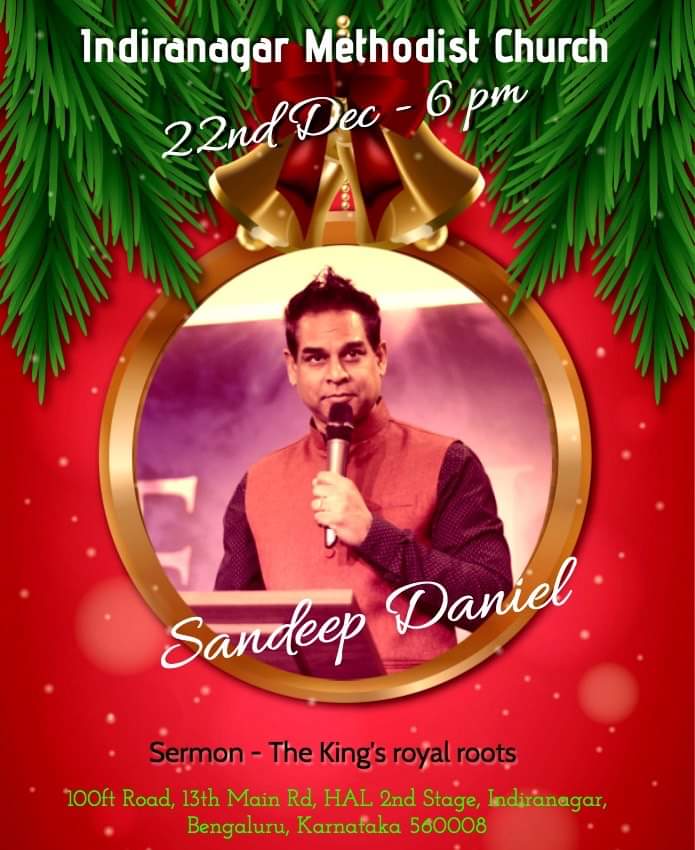The image is an advertisement for an event at the Indiranagar Methodist Church. The background features green pine leaves resembling a Christmas tree, with white spots that look like snowflakes. At the top center, there are red and gold ornaments, including bells and a ribbon. In the middle of the image, a gold-rimmed circle frames a photograph of a man named Sandeep Daniel, whose name is written over the photograph in white text. Sandeep is wearing a reddish-purple shirt with purple sleeves and is holding a microphone, appearing as though he is speaking on a stage. His hair is styled upward in the middle. Above the photograph, in white text, it states "Indiranagar Methodist Church," and beneath that, also in white cursive script, it mentions the event date and time: "22nd December, 6 p.m." At the bottom, in black text, it reads "Sermon: The King's Royal Roots," and below that, the address in smaller, light green text: "100 Feet Road, 13th Main Road, HAL 2nd Stage, Indiranagar, Bengaluru, Karnataka, 560008."